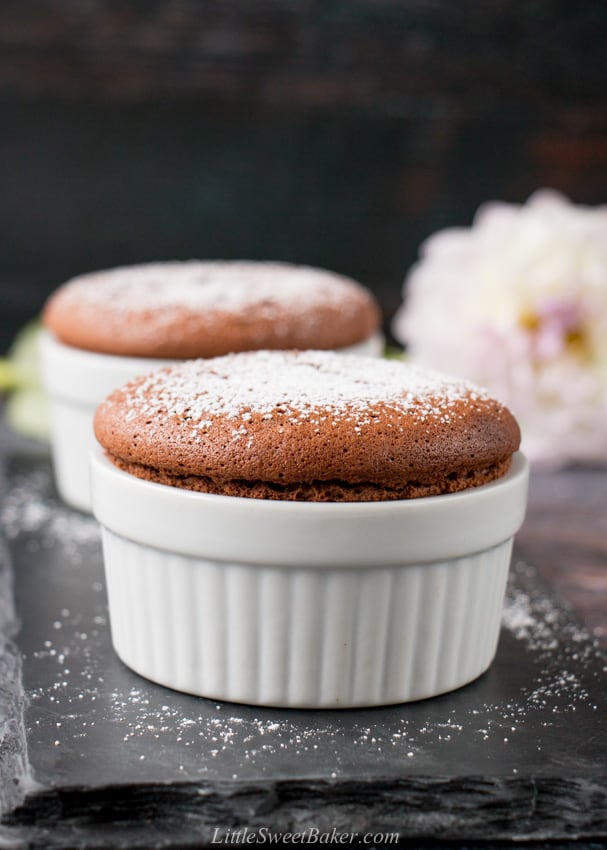In this photo, taken from the website littlesweetbaker.com, there are two white muffin cups, each holding a reddish-brown muffin sprinkled with powdered sugar. The muffins rest on a black stone surface, which also bears a light dusting of powdered sugar. The image’s background is a blurry gray, adding depth while keeping the focus on the muffins. On the right side of the photo, there's a hazy pink and yellow flower, whose soft focus emphasizes the clarity of the muffins. The front muffin is the most prominent, with the second muffin slightly obscured behind it. The black stone surface appears to be placed on a brown table, adding a rustic charm to the composition.